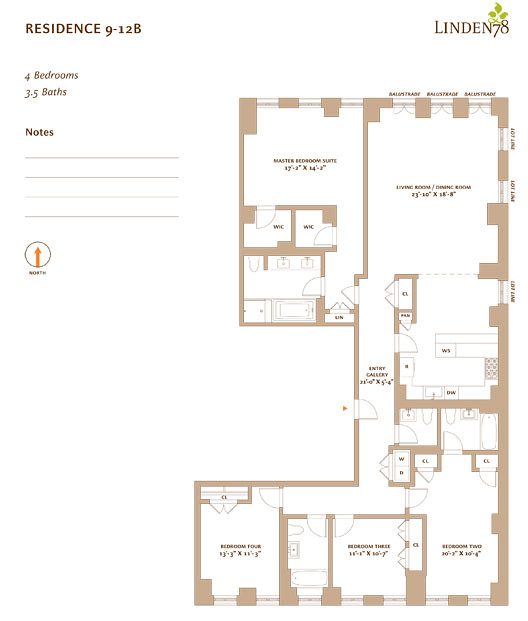This detailed blueprint outlines a single residential unit, possibly an apartment, with the layout filling most of the image and extending to the lower and right edges. The blueprint, depicted in beige, forms a backward "C" shape, indicating an open orientation to the left. Each room is annotated with its intended use and dimensions, although the text is too small to be clearly readable. 

In the upper right corner, a logo reads "Linden 78" in black text, accompanied by a trio of green stylized leaves and a vine above the "78." The upper left corner contains text specifying the unit as "Residence 9-12B," noting it features four bedrooms and 3.5 bathrooms. Below this description, four blank horizontal lines are provided for additional notes, and a round black circle with an orange arrow pointing upward is also present.

The unit appears to include exterior windows, suggesting it is located on the building's periphery, allowing natural light to flow into the rooms.